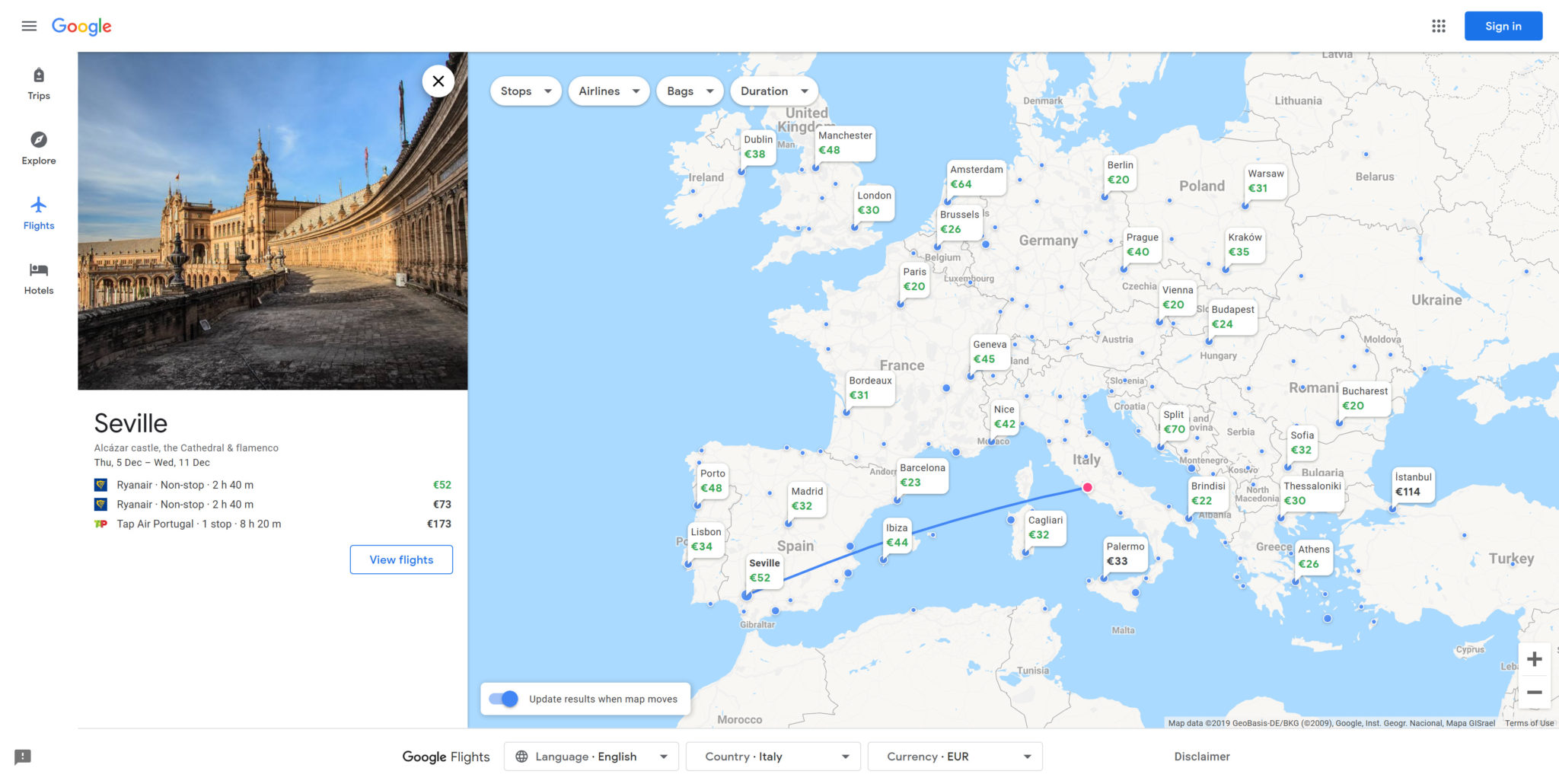This composite image showcases two distinct sections side-by-side. 

On the left side, there is a screenshot depicting a Google search interface. The background is white, and at the top left corner, the iconic multi-colored Google logo is prominently displayed. Along the left margin, there are icons for different sections labeled "Trips," "Explore," "Flights," and "Hotels." In the main section of the screenshot, there is a large color photograph of a historical building set against a clear blue sky. Below this image, the destination "Seville" is noted in bold black text, accompanied by a brief description: "Castle and Cathedral." Travel dates are specified as "Thursday, 5th of December to Wednesday, 11th of December." The section also lists flight options: 

- "Ryanair, non-stop, 2 hours 40 minutes, 52 euros."
- "Ryanair, non-stop, 2 hours 40 minutes, 73 euros."
- "Tap Air Portugal, one stop, 8 hours 20 minutes, 173 euros."

At the bottom of this section, there's a blue button labeled "View Flights."

On the right side of the image, there's a map of Europe. The continents are depicted in white and are labeled with gray or black text. Various flight prices are marked with small white tags, with the costs highlighted in green. This side of the image gives a visual overview of the flight options and their corresponding prices geographically.